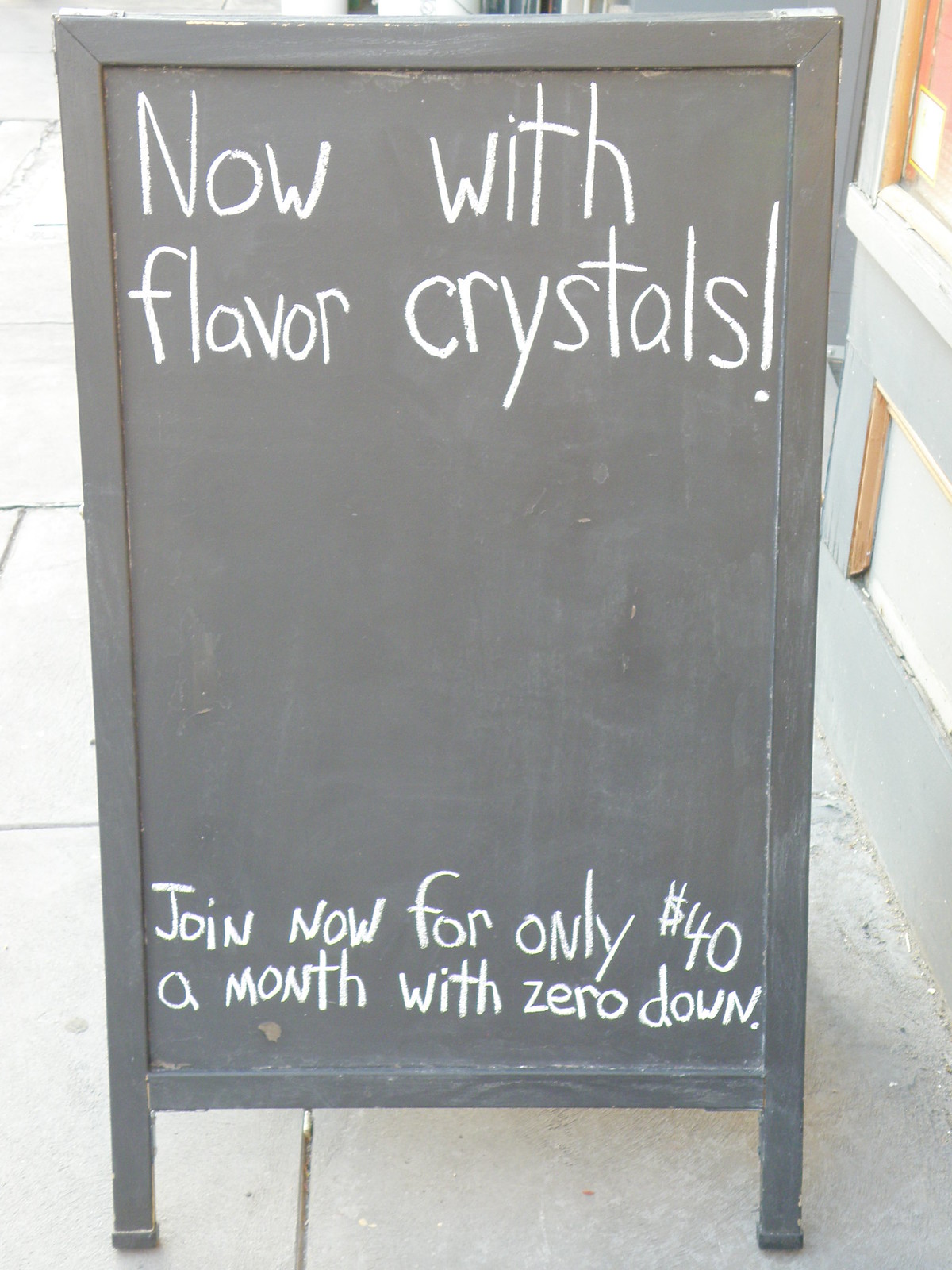The image captures an older, slightly dilapidated A-frame chalkboard standing outside a building on a patio with large cement blocks or bricks underfoot. The black chalkboard, framed in wood, features tidy white chalk writing. At the top, in large letters, it reads, "Now with Flavor Crystals," with smaller text below stating, "Join now for only $40 a month with zero down." The bright, daytime setting reveals the chalkboard positioned near a wooden wall or building exterior, likely suggesting it's outside a coffee shop, wine store, or similar establishment. There is a gap of space in the middle of the chalkboard, possibly intended for future drawings or additional information.